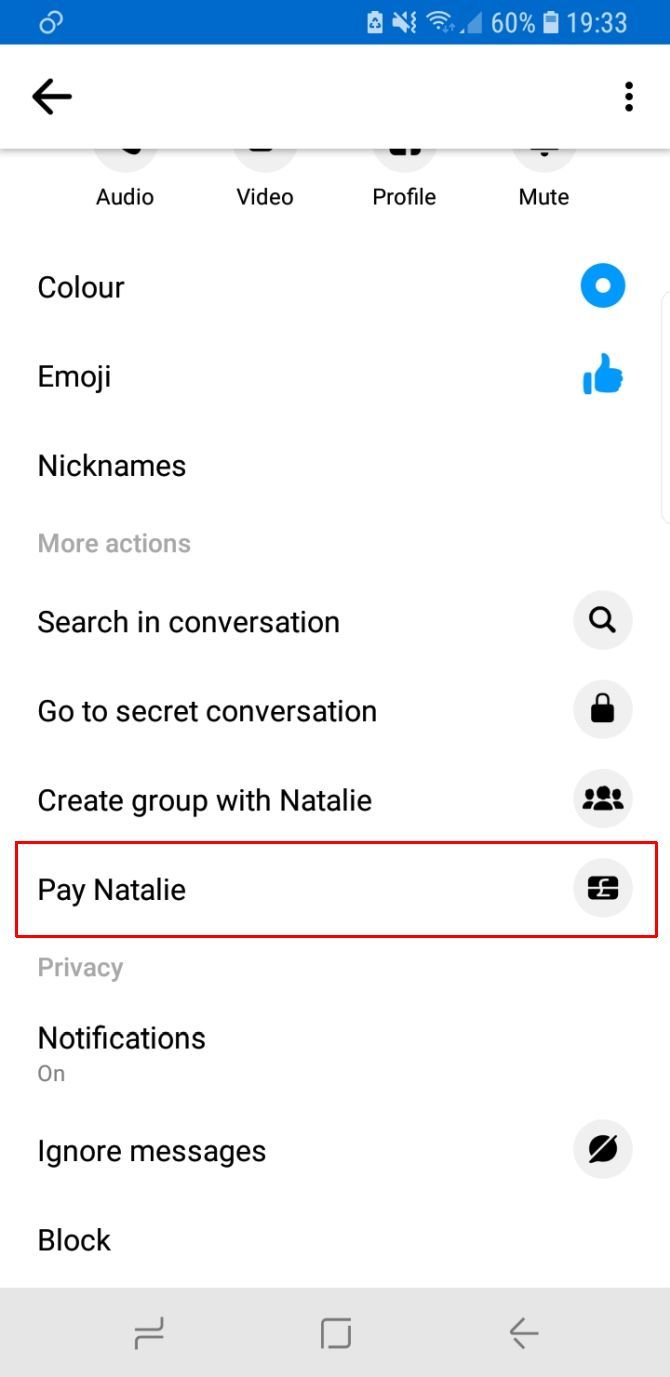Here is the enhanced and detailed caption:

---

The image displays a screenshot taken on a mobile device in portrait orientation, set against a white background. The top of the screen features a cobalt blue bar containing several status icons: the speaker off icon, Wi-Fi signal strength bar, mobile signal bar, and battery charge indicator, which currently shows a 60% charge. The time displayed is 19:33, equivalent to 7:33 PM.

Beneath the blue bar lies a thinner white bar, which includes a left-pointing arrow on the left side for navigating to the previous screen, and a stack of three dots on the right, likely indicating a menu option. Directly below this white bar is a row of spherical icons, labeled as follows from left to right: Audio, Video, Profile, and Mute.

The main content of the screen features about a dozen lines of text, beginning with several settings options. The first line reads "Colour" (spelled "C-O-L-O-U-R," indicating UK spelling) with a blue disc icon to its right. The next line reads "Emoji" followed by a blue thumbs-up icon. Below this is "Nicknames," followed by "More Actions."

Further down, the list continues with "Search in Conversation" paired with a black magnifying glass icon, and "Go to Secret Conversation," which includes a padlock icon. Below is "Create Group with Natalie," accompanied by an icon depicting a group of people. Significantly, "Pay Natalie" stands out as it is selected, surrounded by a red rectangle that spans the entire width of the screen and encloses a pound sterling icon.

The final items listed are "Privacy," "Notifications are on," "Ignore Messages" with adjacent icons, and lastly, "Block."